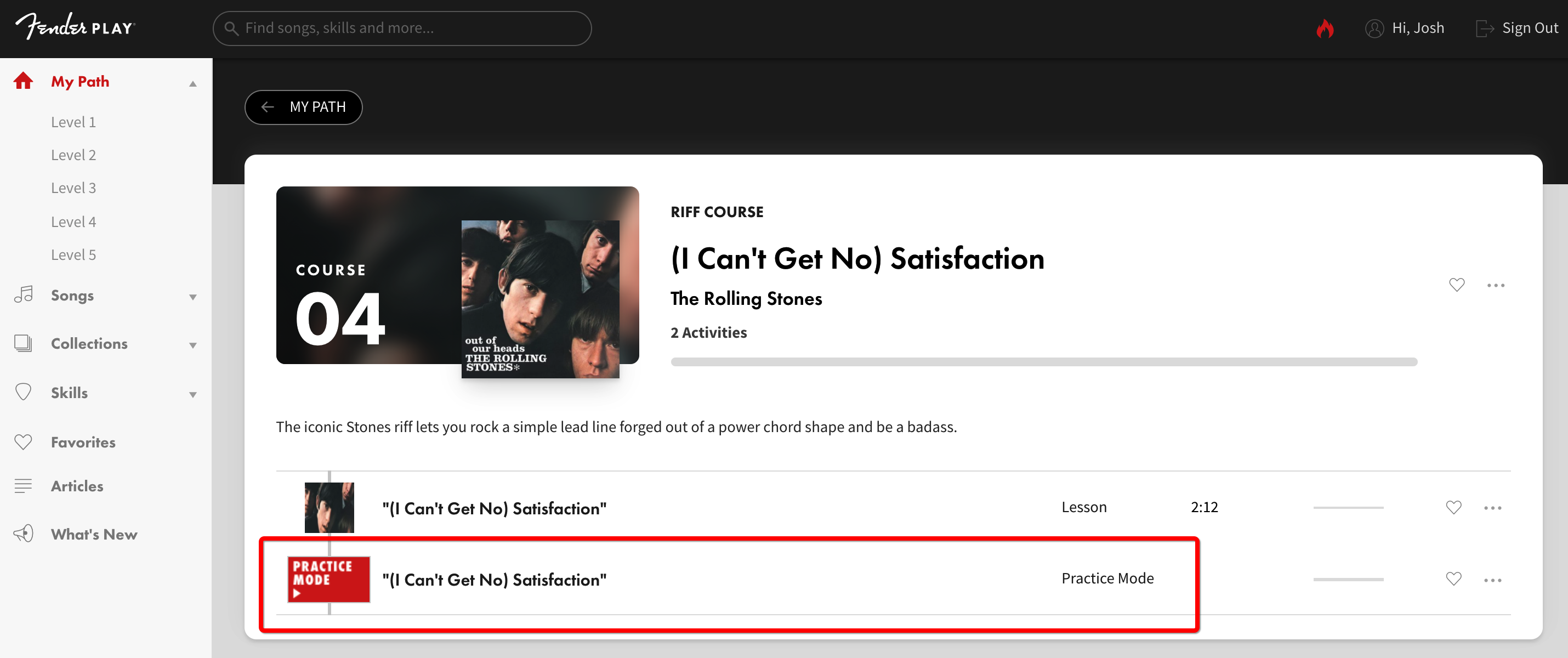In the top left corner of the image, the brand name "Fender" is prominently displayed, followed by the word "Play" in bold text. Adjacent to this, a small image of a red house appears, near which the phrase "My Path" is written in striking red text. Below this section, a series of options are listed: "Level 1," "Level 2," "Level 3," "Level 4," and "Level 5."

The next category headers include "Songs," "Collections," "Skills," "Favorites," "Articles," and "What's New." 

One of the standout elements of the image is a vintage photograph of the Rolling Stones from their early years. Each band member has black hair, and they are all gazing outward together. To the right of this photograph, the caption reads "(I Can't Get No) Satisfaction," followed by "The Rolling Stones" underneath it.

Beside the image, the word "Course" is displayed along with the label "04" beneath it, suggesting a specific course or lesson. The description highlights the iconic Stones riff, noting that it lets players "rock a simple load line, forged out of a paper cord shape, and be a badass." 

Finally, in a red circle, the song title is repeated, and within a red square, the text "Practice Mode" is clearly visible, offering an option for focused practice.